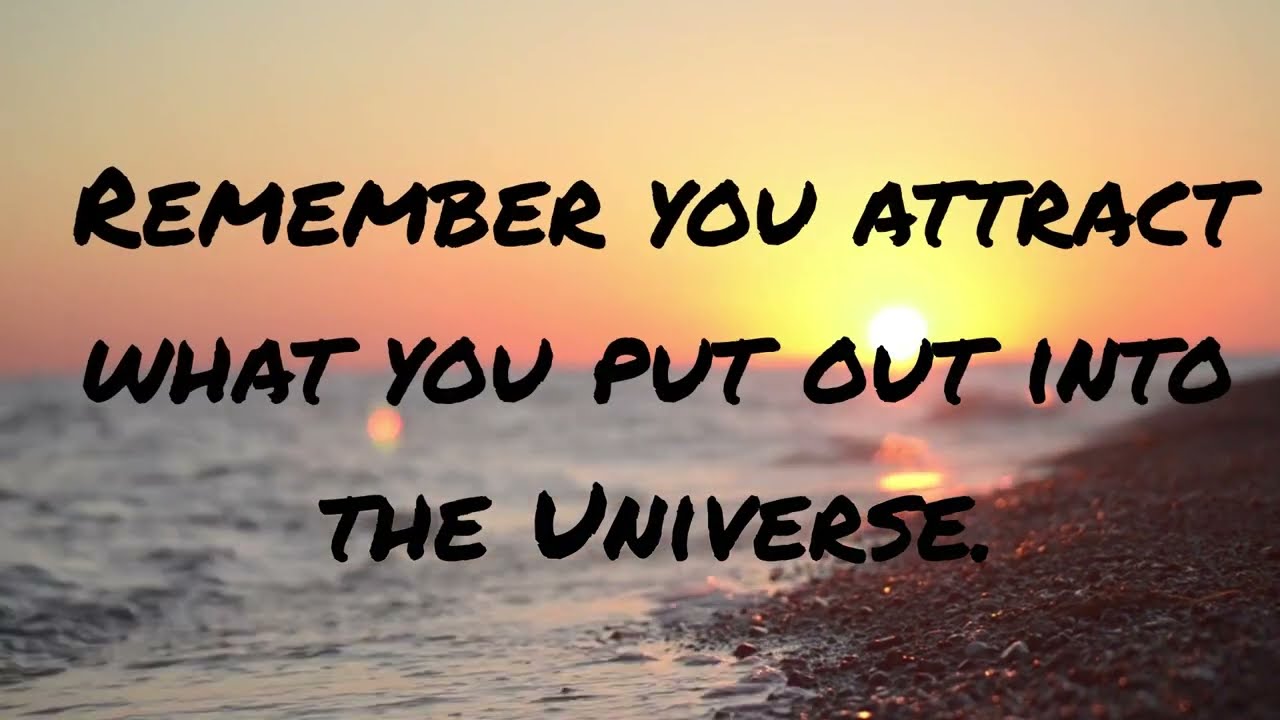The image is a captivating landscape shot taken at sunset, presenting a harmonious blend of natural elements and text. The background depicts a serene water body on the left side, transitioning into a pebbly, reddish sand on the right, where waves meet the shore. The sky above showcases dramatic hues of red and yellow, centered by a brilliant setting sun radiating intense white light. This vibrant scene is accentuated by the reflection of the sun’s red glow on the water, while the sand appears darker due to the diminishing daylight. Superimposed on this tranquil background are three lines of text in uneven black capital letters resembling handwritten marker strokes: "REMEMBER YOU ATTRACT WHAT YOU PUT OUT INTO THE UNIVERSE." The sun aligns with the second line of the text, subtly illuminating the message. The overall composition conveys a powerful visual and textual reminder, set against the natural beauty of a sunset beachscape.